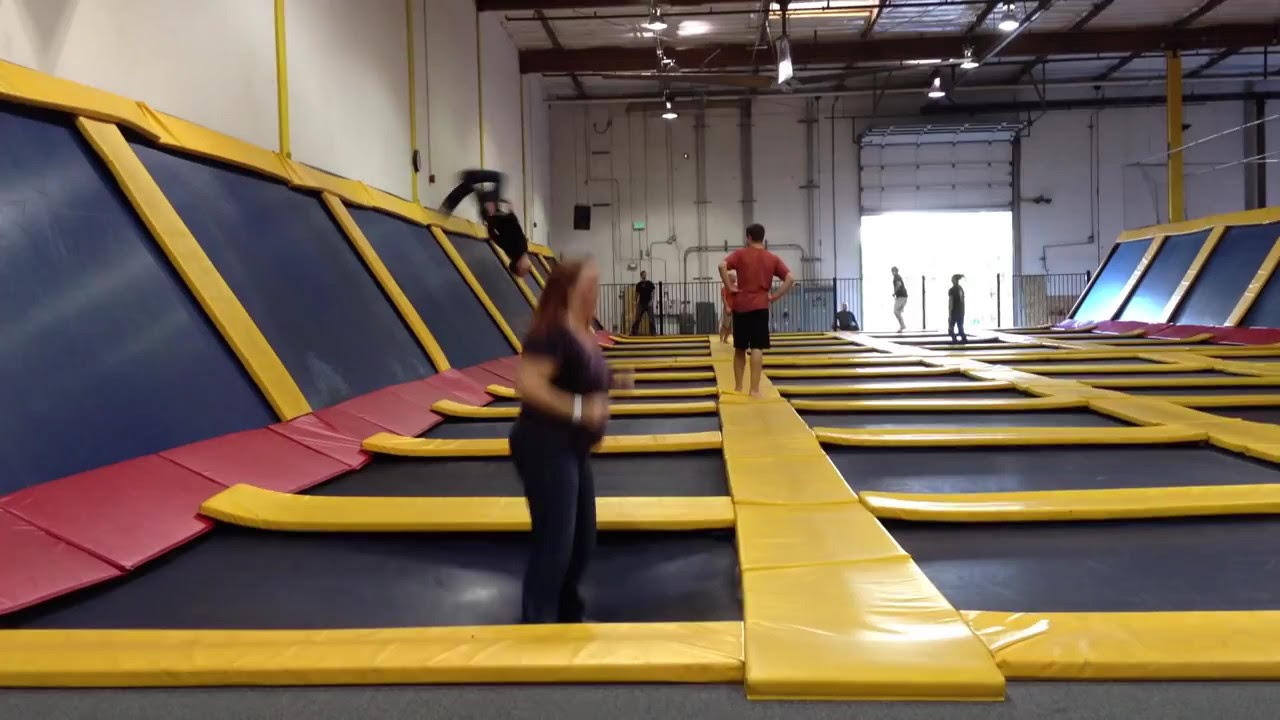The image depicts the interior of a large trampoline park that resembles a gymnasium or a warehouse with a high ceiling and big metal walls. A prominent feature is a large garage door, three-quarters open, letting in bright daylight and silhouetting two people standing near it. The floor is covered with blue and yellow mats, where the blue sections appear to be the trampoline surfaces and the yellow parts serve as walkways connecting different jumping areas. 

In the foreground, a woman in a purple t-shirt and blue jeans is jumping on a bluish-black trampoline mat. To the left, she points towards the right as she leaps. Behind her, a young man in a red t-shirt and black shorts watches another young man in all-black attire executing a somersault mid-air. Additional people can be seen further in the background, engaging and observing the lively environment. The walls of the building are lined with mats arranged diagonally in blue and yellow, reinforcing the vibrant and energetic atmosphere of the trampoline park.